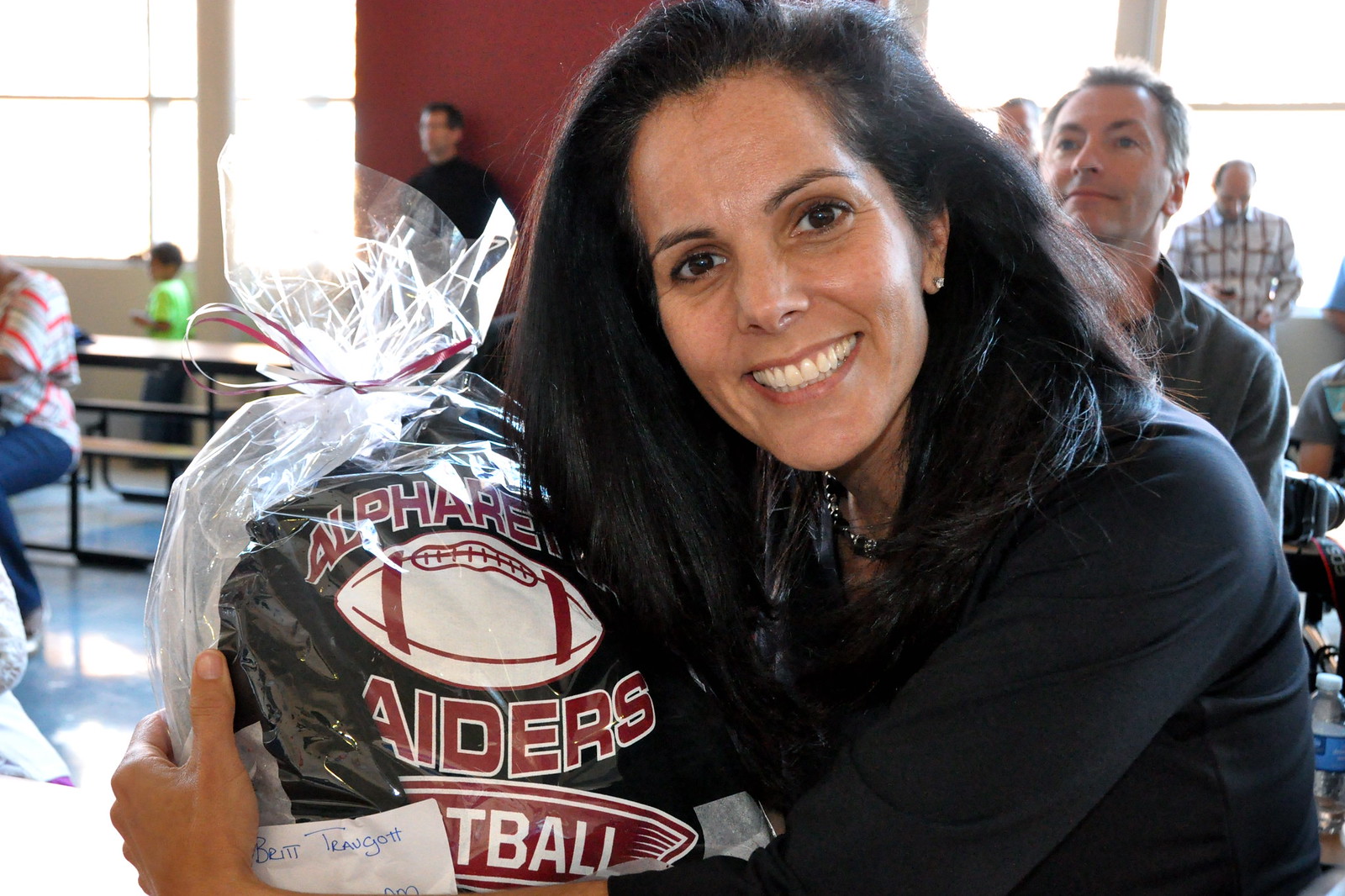In the wide rectangular photograph, a woman with voluminous dark brown hair is positioned on the right side, facing forward and smiling broadly, showcasing her teeth. She has a fair, tan complexion and is wearing a detailed outfit that includes a black shirt layered under a long sleeve brown shirt, a black necklace, and diamond earrings. In her right hand, she holds a clear plastic bag containing a black and red football jersey, which is emblazoned with the logo of the Alpharetta Raiders—featuring maroon text with a white border and an image of a red and white football at the center. There is a ribbon around the cellophane-wrapped bag. The background reveals a school cafeteria setting with windows letting in sunlight, a red wall, and several long tables. A man in an olive sweater is partially visible behind her, looking up.